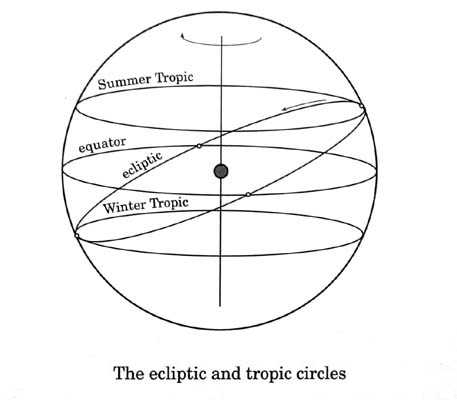The image depicts a black-and-white diagram illustrating the ecliptic and tropic circles, set against a white background. At the center of the large, round black circle is a smaller black dot with a vertical line running through it, possibly indicating the Earth's core. Inside the large circle, there are several smaller rings positioned both horizontally and diagonally. The topmost ring on the diagram is labeled "Summer Tropic," and the bottom-most is labeled "Winter Tropic." Between them is a horizontal ring labeled "Equator." A diagonal line, indicating the ecliptic, connects the left edge of the Winter Tropic to the right edge of the Summer Tropic, intersecting parts of the Equator. The labels are written in a traditional serif style font. At the bottom of the image, it is stated that this is a diagram of the ecliptic and tropic circles, implying the depiction of the Earth's rotational dynamics or related celestial mechanics.